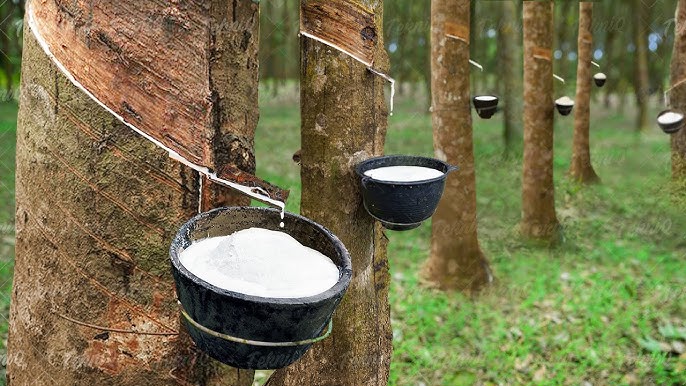In this detailed outdoor photograph set in a woodland area or tree farm, a row of evenly spaced trees extends into the background. Each tree features a distinct diagonal cut near its trunk, facilitating the flow of sap. Attached to each of these trees by white rope or twine is a small, black bucket, positioned to catch the milky-white liquid sap dripping from the cuts. The forest floor, composed of grass interspersed with patches of dirt, occupies the lower three-fourths of the image. In the top fourth, a background of additional trees is visible, though they are out of focus. This orderly arrangement of trees and buckets suggests an organized process of sap extraction, with six such setups clearly visible in the foreground. The entire scene captures the essence of a structured operation within a natural, wooded environment.